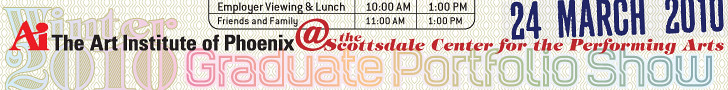The image depicts a thin, rectangular poster featuring a patterned white background with circle line designs resembling a beehive. At the top-right corner, in blue, it states "24 March 2010." Centered below, bold red letters display "AI," the emblem of the Art Institute of Phoenix. Following this, in black text, it reads "The Art Institute of Phoenix at the Scottsdale Center for the Performing Arts."

The key event, highlighted as the "2010 Graduation Portfolio Show," is prominently mentioned. Below this central heading, details such as "Employer Viewing and Lunch 10 a.m. to 1 p.m." and "Friends and Family 11 a.m. to 1 p.m." appear in small black print. The date and time details are also colored, featuring a rainbow gradient of pink, orange, blue, and green. The left side of the banner subtly includes "Winter 2010," styled with a faded gradient look.

Overall, the small yet distinctly designed poster neatly combines informative text with vivid color accents to announce the Art Institute of Phoenix’s Graduate Portfolio Show event on March 24, 2010, at the Scottsdale Center for the Performing Arts.